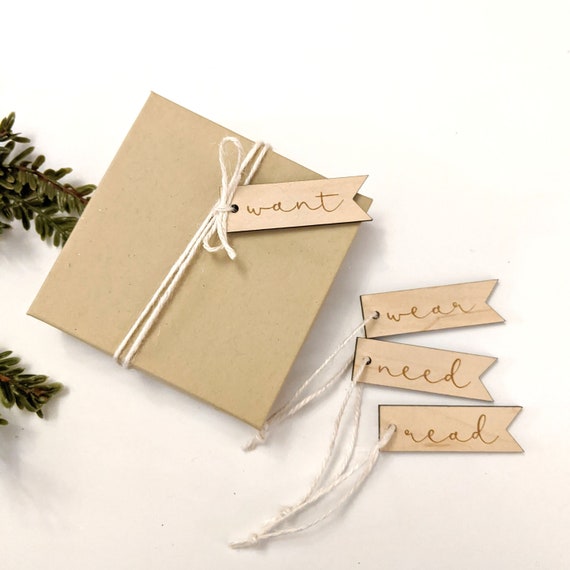The image features a square-shaped cardboard box, which appears to be a gift, wrapped in brown paper and white string that is tied into a bow. A tan tag is attached to the bow with a handwritten word "want" in gold cursive. In the upper left and middle left sections of the image, small leaves or pine needles are visible, attached to branches that stick out. The background of the image exhibits a gradient, transitioning from white at the top to beige at the bottom. To the right of the box, three additional tags with strings lie on the surface. These tags read "wear," "need," and "read." Each tag has a hole at one end for the string and a V-shaped cut on the opposite end.